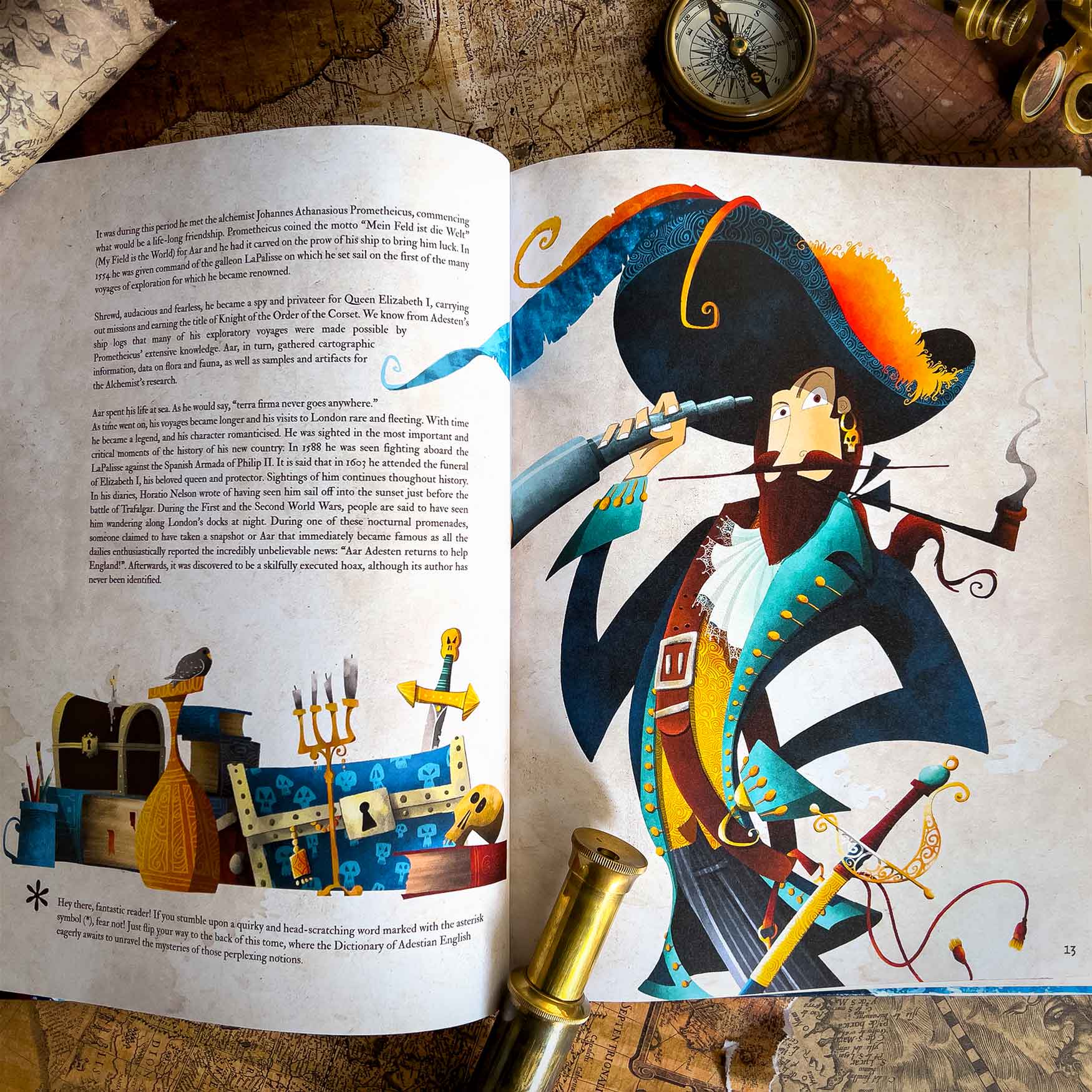The picture features an open children's storybook, displaying two distinct and colorful pages. The left page showcases three paragraphs of unreadable, small black text, followed by an illustration of pirate treasure, including several treasure chests, a candelabra, a skull, a sword, a book, a cup containing writing implements, and additional books. The right page prominently features an intricately detailed drawing of a bearded pirate. He dons an elaborate dark blue hat adorned with orange and blue feathers, a blue jacket with light blue lapels, frills around his neck, and a belt tied like a banner. He holds a silver telescope and smokes a pipe, with a sword at his side. The jacket reveals hints of yellow clothing underneath. In the background, there are various maps and a compass. The image brims with a mix of vibrant colors, including yellow, red, blue, black, and gold.